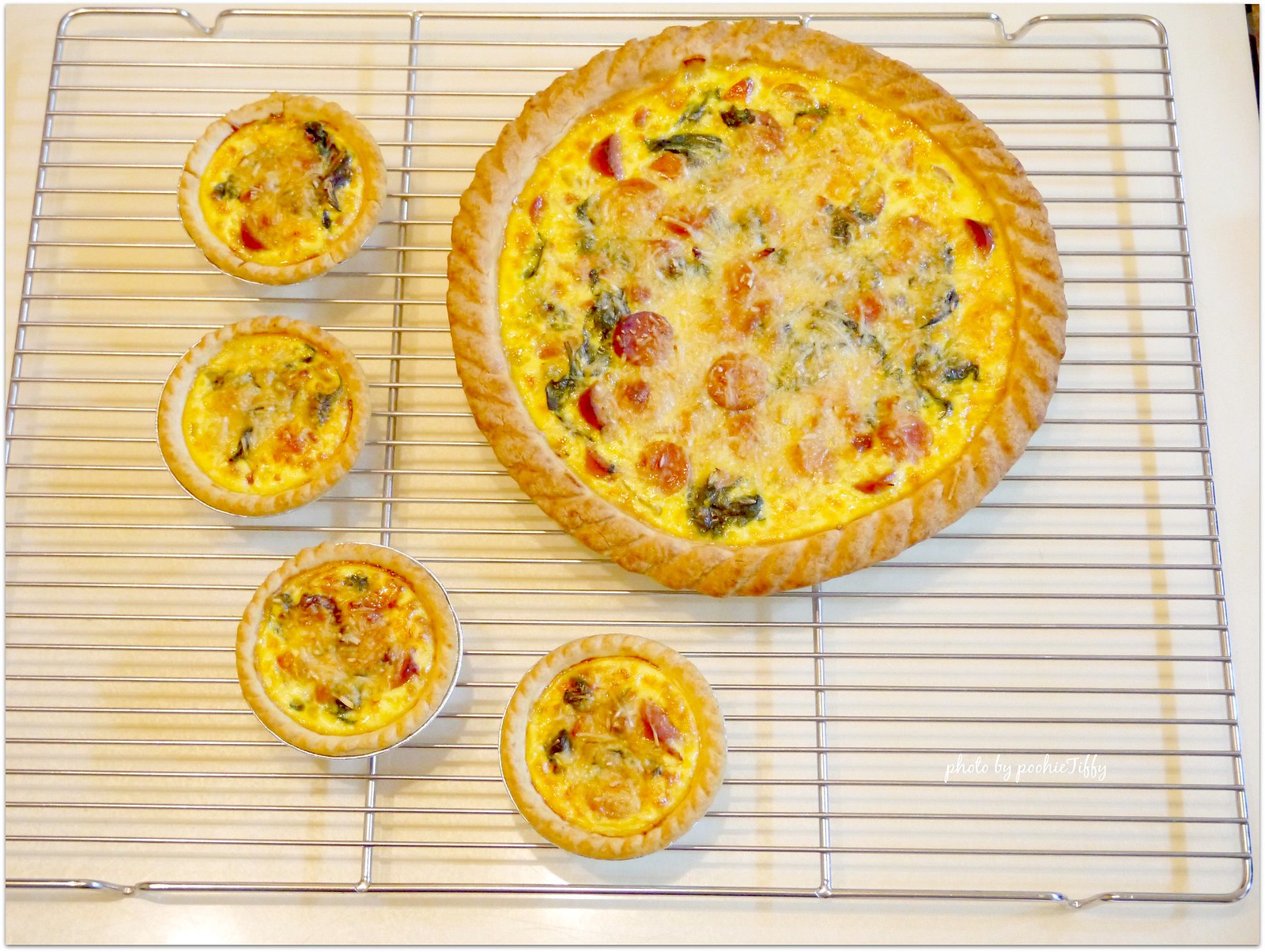The image features an assortment of quiches, with one full-size quiche positioned to the right and four mini quiches forming a semi-circle to its left. Each quiche showcases a golden-brown, crispy homemade crust and is filled with a delectable mixture of egg, cheese, spinach, and some variety of meat, possibly pepperoni. The quiches have just been pulled from the oven and are now cooling on a metal wire rack, which casts detailed shadows onto the white counter beneath. The counter sports a white towel with widely spaced yellow lines. Light enters from the top, adding depth to the cooling rack’s shadows. Additionally, a faint watermark reads "photo by Peachy" in small, light script.